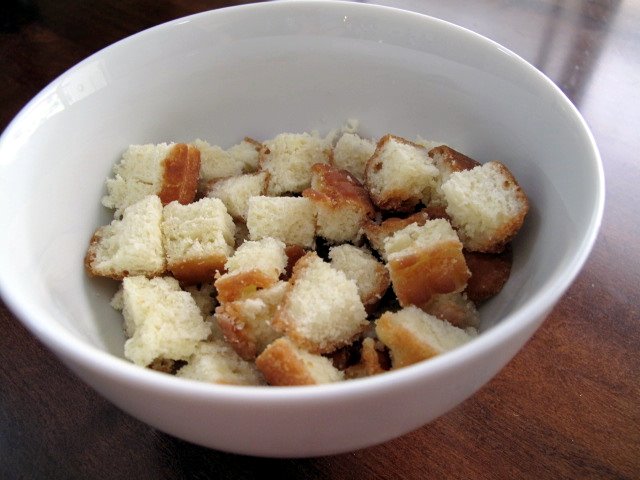The image is a well-lit, indoor color photograph showcasing a white porcelain bowl filled with fresh, fluffy bread cubes, likely intended for croutons or stuffing. The bowl, measuring approximately seven to eight inches in diameter, contains around 35 to 40 bread cubes, filling it about halfway. Each cube displays a golden brown crust on the outside and white, soft interior. The bowl is placed on a polished, dark cherry wood table, notably reflecting light on the top right corner of the image, while the upper left and lower left corners of the background appear dark. Shadows cast inside the bowl add depth to the composition, and despite a slight angle in the view, the image remains sharp and detailed, with no words or text present.